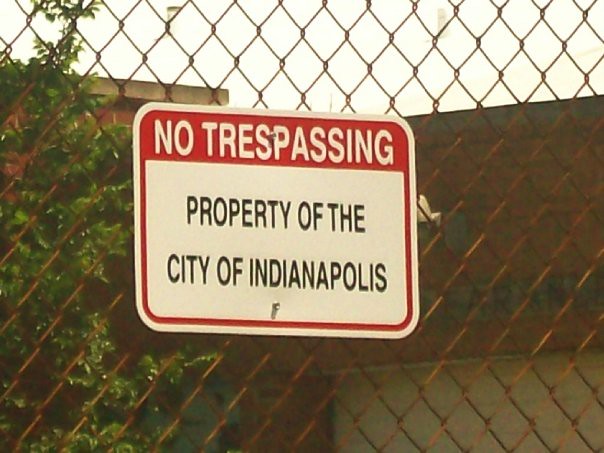This image captures a chain-link fence with a slightly rusty, brownish tint prominently in the foreground. Centrally mounted on the fence is a rectangular sign with a bold red border, within which the phrase "NO TRESPASSING" is emblazoned in all caps with white text on a red background. Below this warning, the sign continues in a white section with the declaration "Property of the City of Indianapolis" in black letters, imparting a serious tone regarding trespassers. Behind the fence, on the left side, a verdant tree with vibrant green leaves stretches vertically, almost reaching the top of the image. To the right of the tree, partially obscured, stands a dark brick building, its subtle details like dark windows and a large off-white section, possibly a garage door, faintly visible. Above both the sign and the tree, the top edge of the building can be seen, characterized by a gray concrete rooftop border.